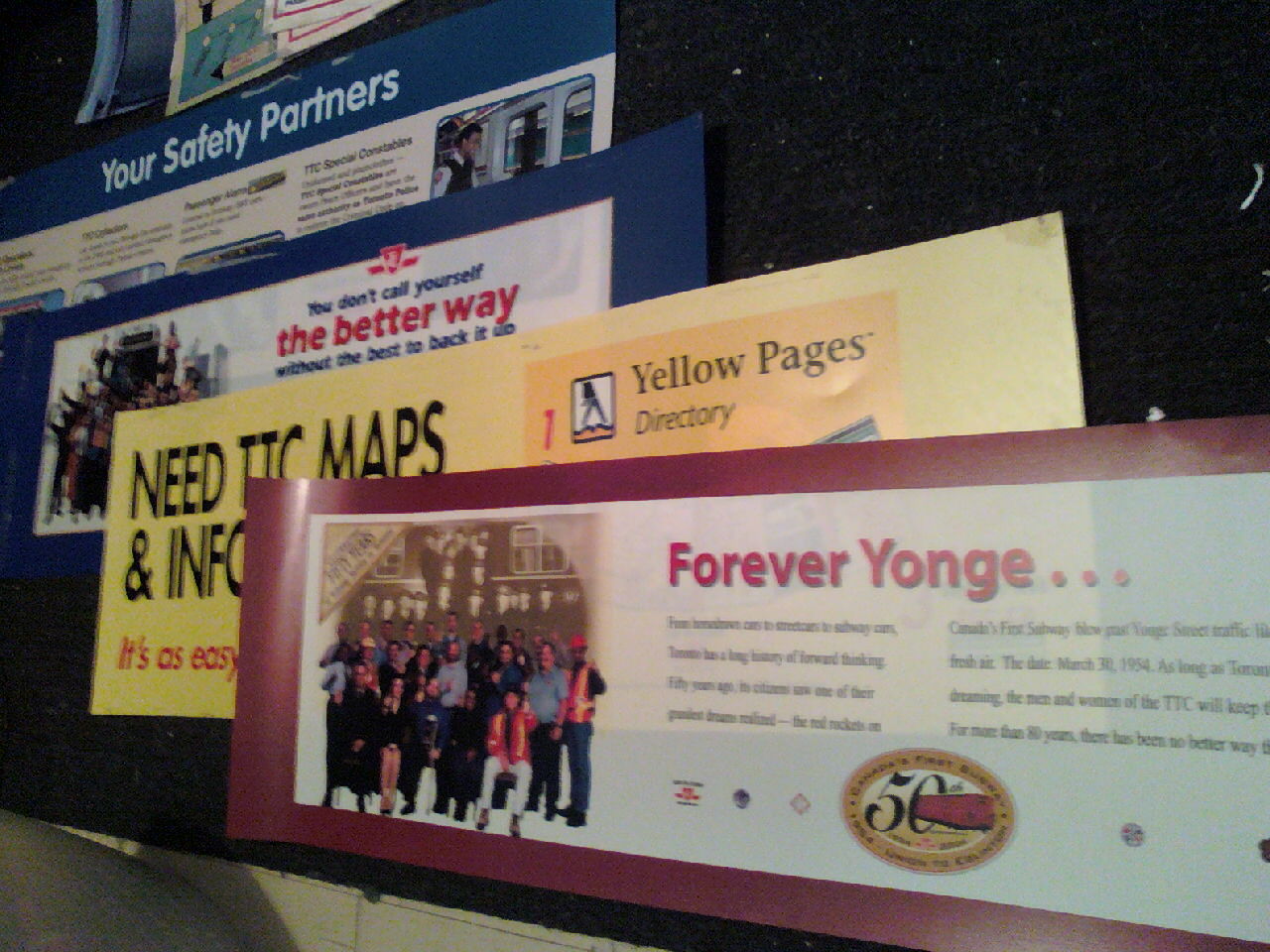The image depicts a black bulletin board adorned with several colorful signs arranged in a staggered, almost staircase-like fashion. The topmost sign is pink and white with red accents, prominently displaying "Forever Yonge" with "Yonge" uniquely spelled y-o-n-g-e. It features a photograph of a diverse group of people in various uniforms, suggesting a celebratory theme, underscored by a gold oval with "50th" inscribed in it. Below this is a yellow sign with text partially visible, mentioning "Yellow Pages Directory" and information about maps. Further down is a blue sign stating, "You don’t call yourself the better way without the best to back it up." At the bottom is another blue notice with "Your Safety Partners" framed by a blue outline. Despite the overall blurriness of the image, these distinct elements each advertise different services and appear to be well-organized on a primarily black surface.